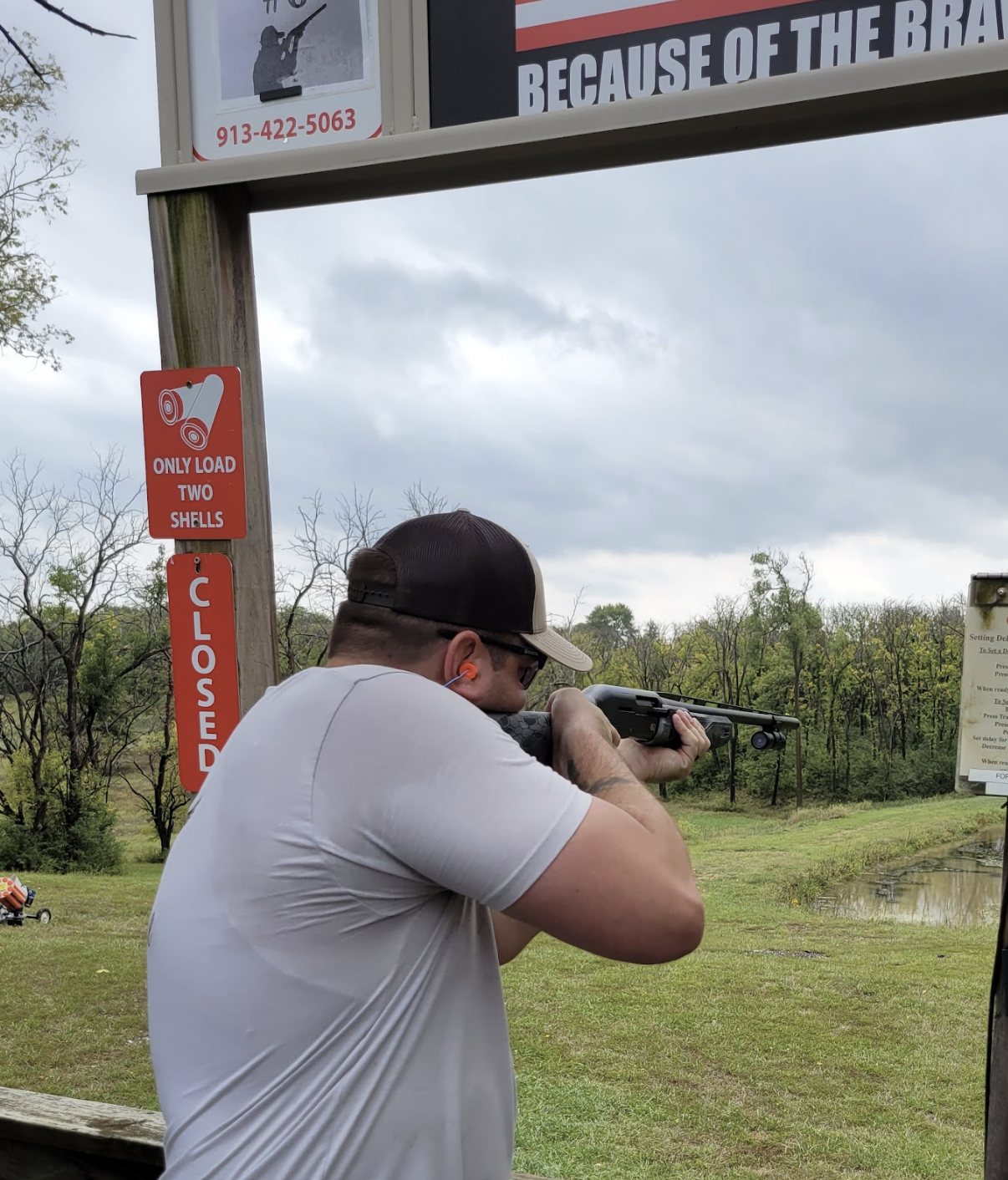In this detailed image taken at an outdoor shooting range, a man stands in a framed archway with multiple signs around it. He's wearing a gray t-shirt and a black cap, and he has orange earplugs for hearing protection. The man is aiming a pump-action shotgun with no scope, looking directly ahead and pointing the barrel to the right side of the image. 

He's positioned next to wooden posts that bear several signs, including one stating "Only Load Two Shells" and another indicating "Closed." There's also a visible phone number and additional warning signs attached to the structure. In the background, the freshly mowed green grass extends to a pond, beyond which are trees just starting to sprout leaves, suggesting an early spring setting. On the left side of the image, there's a clipboard hanging on the framing structure and a wheeled cart carrying orange cylinders.

The overall scene depicts a typical shooting range environment, with signs ensuring safety and protocol adherence, and the natural surroundings indicating a well-maintained outdoor area.